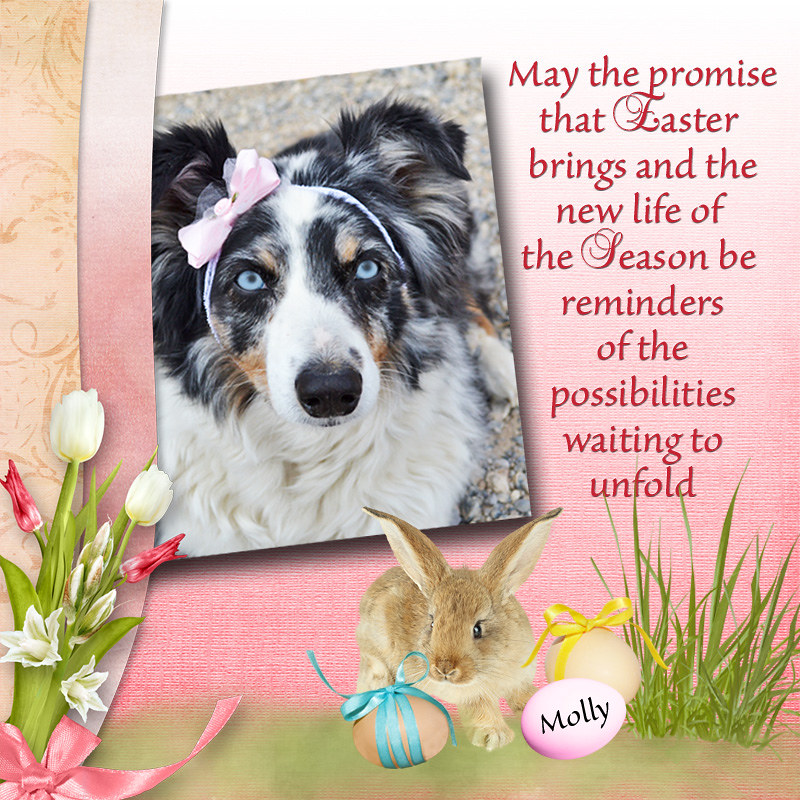The image is a vibrant Easter-themed inspirational graphic with a dominant pink background. At the center, there's a large, clear photo of an Australian Shepherd dog with striking blue eyes, a black and white fur coat, and a distinctive pink bow around its head. The dog’s chest is predominantly white, and it has a black nose, looking endearingly up at the viewer. Surrounding the dog are delicate white and pink tulips, a cheerful bunny rabbit next to a patch of grass, and several Easter eggs adorned with ribbons, one of which bears the name "Molly." The composition includes a combination of pink and beige margins on the sides and a greenish fade at the bottom. The right side of the image features an inspirational message in red script: “May the promise that Easter brings and the new life of the season be reminders of the possibilities waiting to unfold.” The overall aesthetic of the card is serene and pastel, capturing the hopeful spirit of Easter.